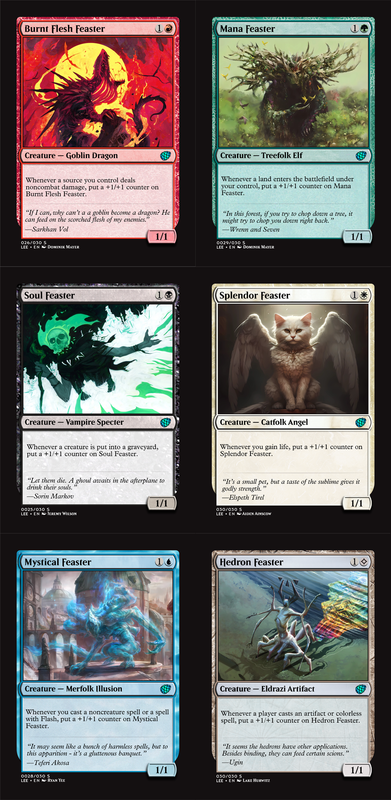This image displays six unique cards from a battle-style card game, each featuring a distinct creature. At the top left is the "Burnt Flesh Eater," a red card representing a fearsome creature described as a Goblin Dragon, with a spiked back and a large open mouth. To its right, a green card labeled "Mana Feaster" depicts a hybrid of a tree and person, categorized as a Treefolk Elf.

Below, the "Soul Feaster" card features a Vampire Specter with a ghostly appearance and a green skull, hovering menacingly. Adjacent to that is the "Splendor Feaster," showcasing a mystical blend of an angel and a cat. Further down is the "Mystical Feaster," a blue card depicting a crouching Merfolk Illusion creature. On the far right, the "Hedron Feaster" card presents a formidable entity resembling a spider with multiple legs and a human body, designated as an Eldrazi Artifact. Each card is richly illustrated to capture the unique essence and abilities of the creatures in this captivating card game.